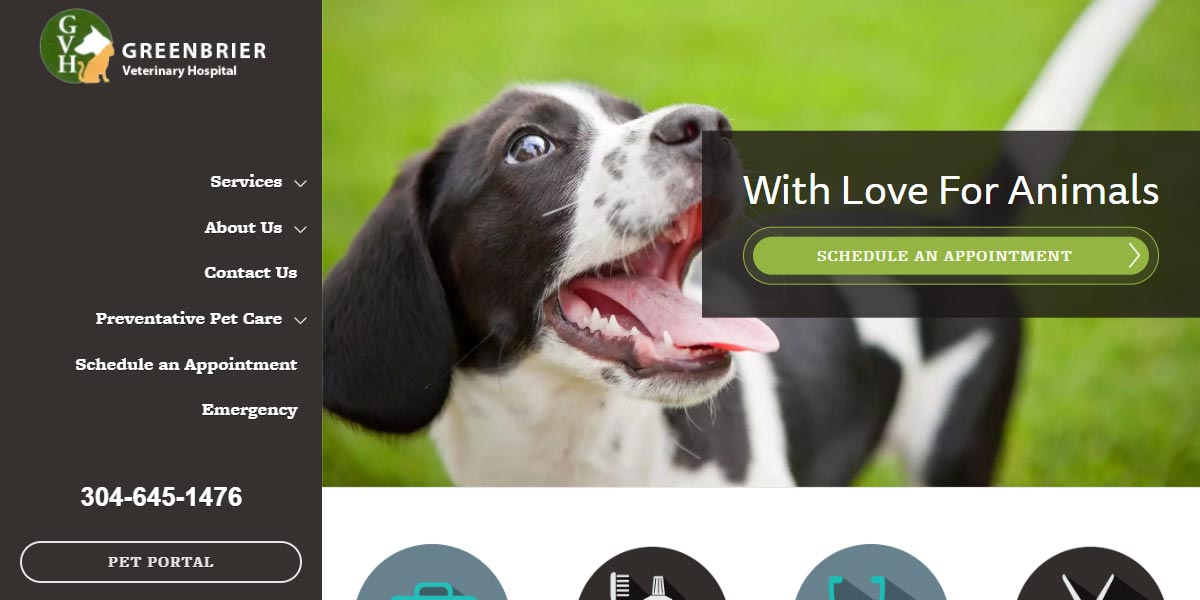This is an image of a website dedicated to animal care, specifically for the Greenbrier Veterinary Hospital. prominently displayed in the upper left corner is a blue icon incorporating the letters "GVH" arranged vertically, with the depiction of a dog's head partially overlaid by a cat's neck. Adjacent to this icon, the text "Greenbrier Veterinary Hospital" is clearly visible. Beneath the heading, there are several drop-down menu options listed: Services, About Us, Contact Us, Preventative Pet Care, Schedule an Appointment, and Emergency. 

A contact phone number, 304-645-1476, sits underneath these menu options, followed by an oval-shaped button labeled "Pet Portal" against a black background. The central section of the page features a prominent image of a small, black-and-white dog with brown eyes and an open mouth, revealing its tongue. The dog appears to be gazing upwards, with its right eye in clear view against a faded green backdrop. Toward the bottom of the page, some circular icons in gray and black are present but indistinct. Text below the dog reads "With Love for Animals," emphasizing the website's theme of compassionate animal care.